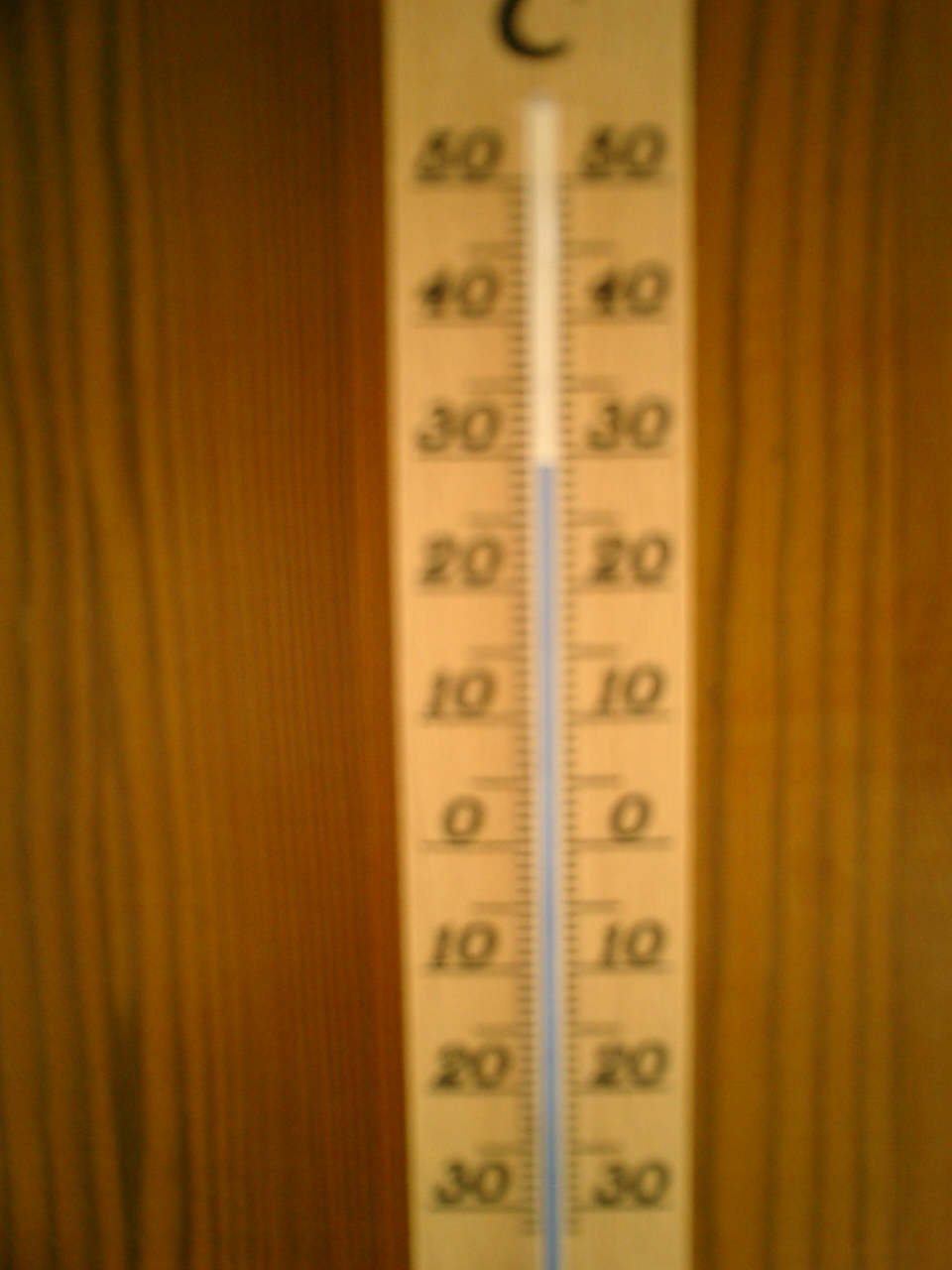A blurred image showcases a white thermometer mounted on a light brown wooden panel with darker streaks. The thermometer, featuring a central blue liquid column, ranges from -30°C to 50°C. Numbers are marked in black on both sides of the scale: -30, -20, -10, 0, 10, 20, 30, 40, and 50. The top of the thermometer, slightly cut off, reveals a blue "C" indicating Celsius. The bottom part is also not visible, lacking a bulb, with the blue liquid extending downwards. The wooden panel's texture displays pronounced black lines, especially towards the edges, adding to the intricate background. The thermometer reads 30 degrees Celsius, despite the overall image being out of focus and relatively light in brightness.